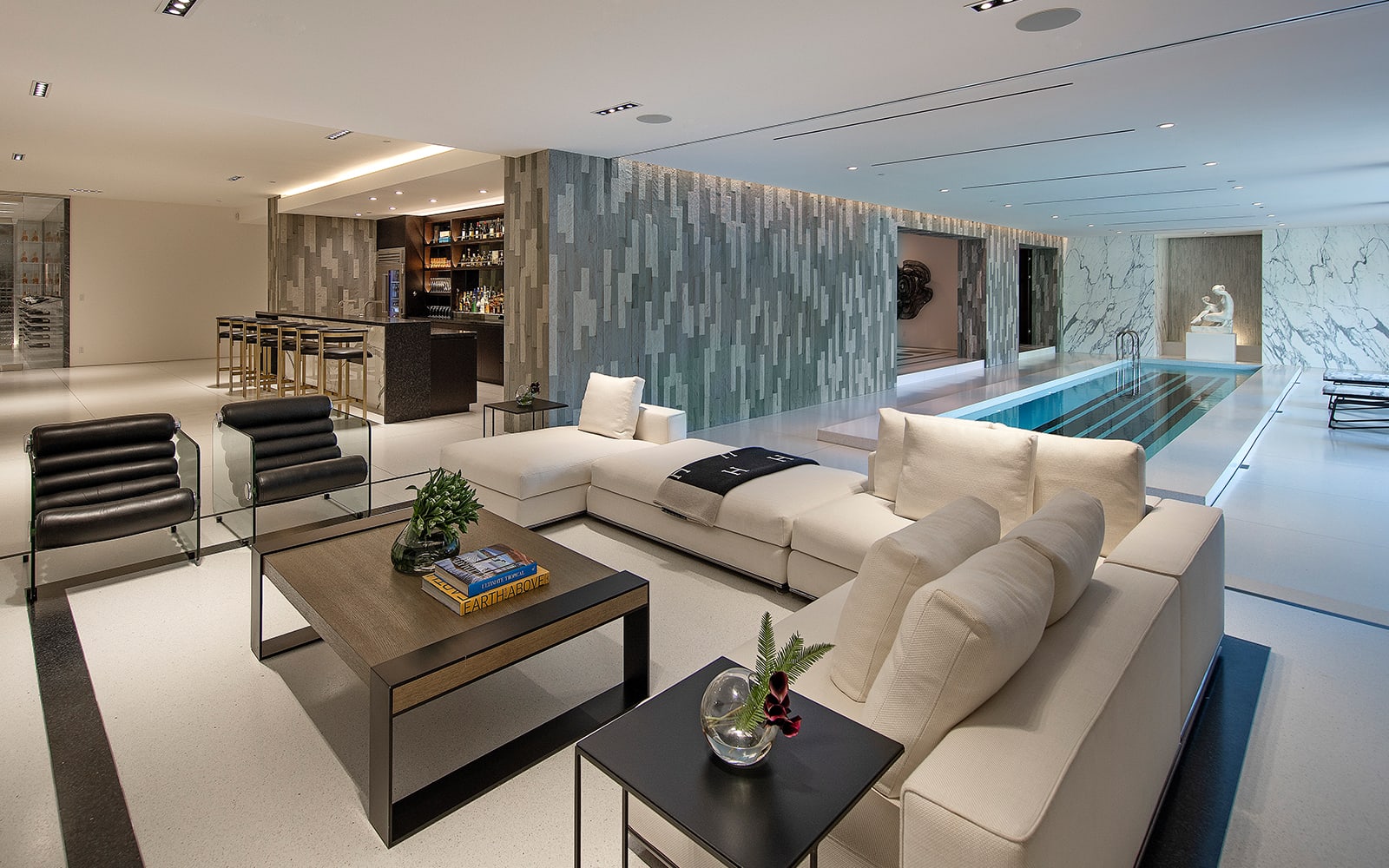This detailed photograph captures an elegant, luxurious interior that could belong to a high-end hotel or the home of someone affluent. The central focus is a sunken living room featuring a white sectional couch adorned with a sophisticated Hermes blanket. On either end of the couch are sleek black tables. A brown wood coffee table in front supports two books and a small plant, adding to the room's tasteful decor. Two modern black chairs with clear glass sides flank the coffee table. The setting is bordered on the left by a bar area with several stools, and shelves stocked with liquor bottles, suggesting a space designed for entertaining. The walls showcase a distinctive abstract pattern in shades of dark and light gray. To the right, a small, blue dipping pool is visible, complete with metal ladder rungs and capped off by a striking white stone sculpture at its far end. This stylish environment, perfectly staged and immaculately detailed, appears ready for a high-end real estate listing or a feature in a luxury magazine.